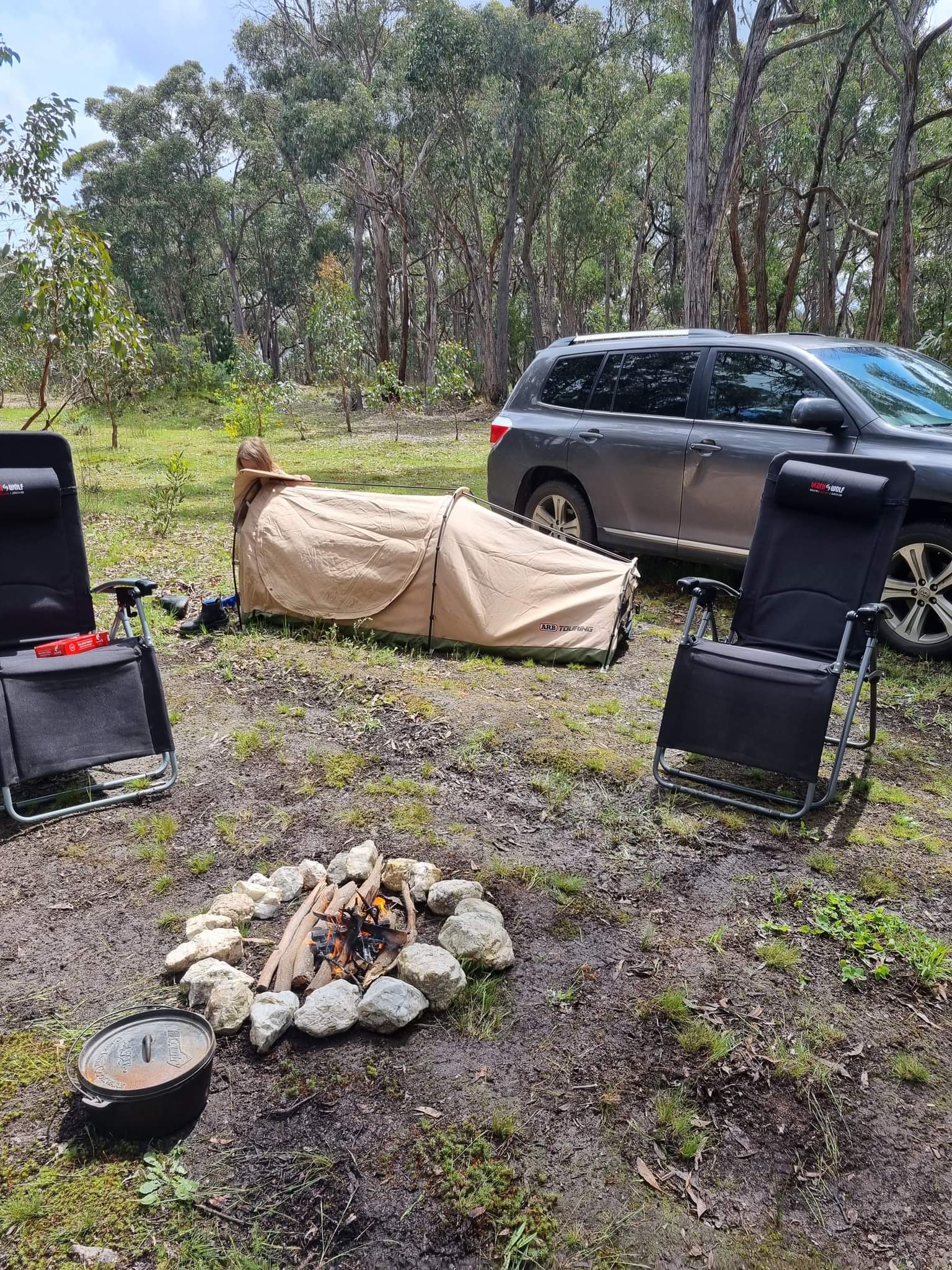The image depicts a detailed camping scene set in a wooded area with tall trees. At the center of the campsite, a small campfire burns brightly within a circle of light gray and white hand-sized stones. Nearby, a cast iron Dutch oven, slightly rusted on the lid, sits to the bottom left of the campfire, suggesting it is used for cooking. Surrounding the fire are two comfortable black zero gravity chairs, one of which has a red package placed on it. Positioned behind the chairs is a small, low-to-the-ground tent made of tan fabric with a dark green base. The tent's entrance is flanked by a pair of boots, and partially visible inside is a person with blonde hair. A gray SUV, possibly a Toyota, is parked behind the tent. The ground around the campsite is a mix of dirt with patches of green grass and moss, while the background reveals a serene forest with tall trees, their foliage concentrated high above.